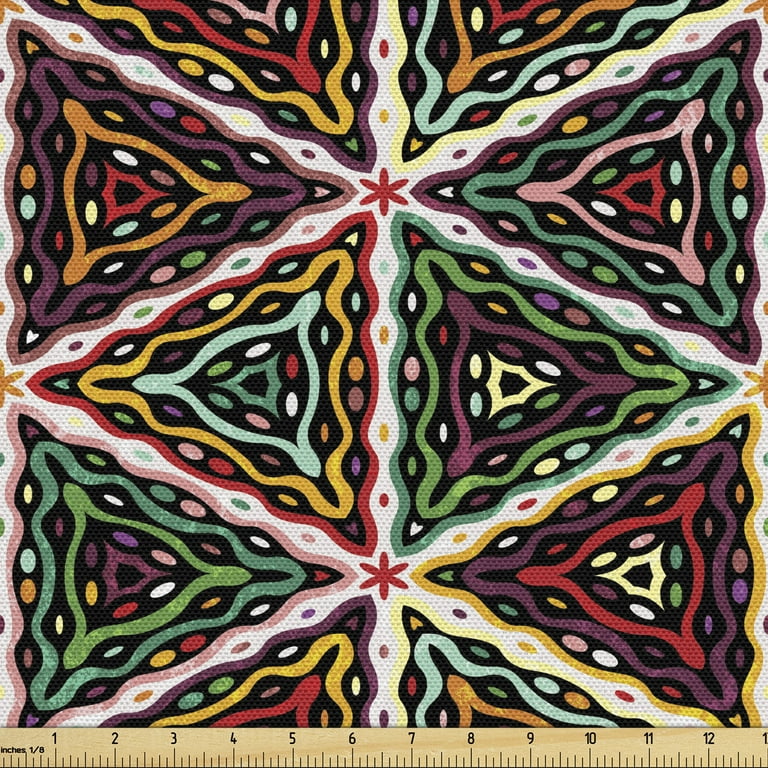This is a vertically rectangular, handmade painting on canvas, likely created using watercolors and bold black ink. The bottom of the image features a beige ruler marked in inches, up to 13 inches, providing a size reference. The painting showcases a series of geometric shapes organized around diagonal and vertical white lines that create a diamond pattern at the center, sectioning off numerous colorful triangles. Inside the diamond, nested irregular triangles of green, pink, and dark red culminate in the center. These triangles are set against a backdrop of repeated patterns in varying colors, including dark purple and dark green triangles elsewhere in the image. Small, colorful oblong dots, including pastel hues like white and red, are scattered throughout the triangles, as well as within the white lines. At the intersections of the white lines, vibrant red stars can be seen. The entire composition is vibrant and dynamic, illustrating a meticulous and thoughtfully executed piece of art.